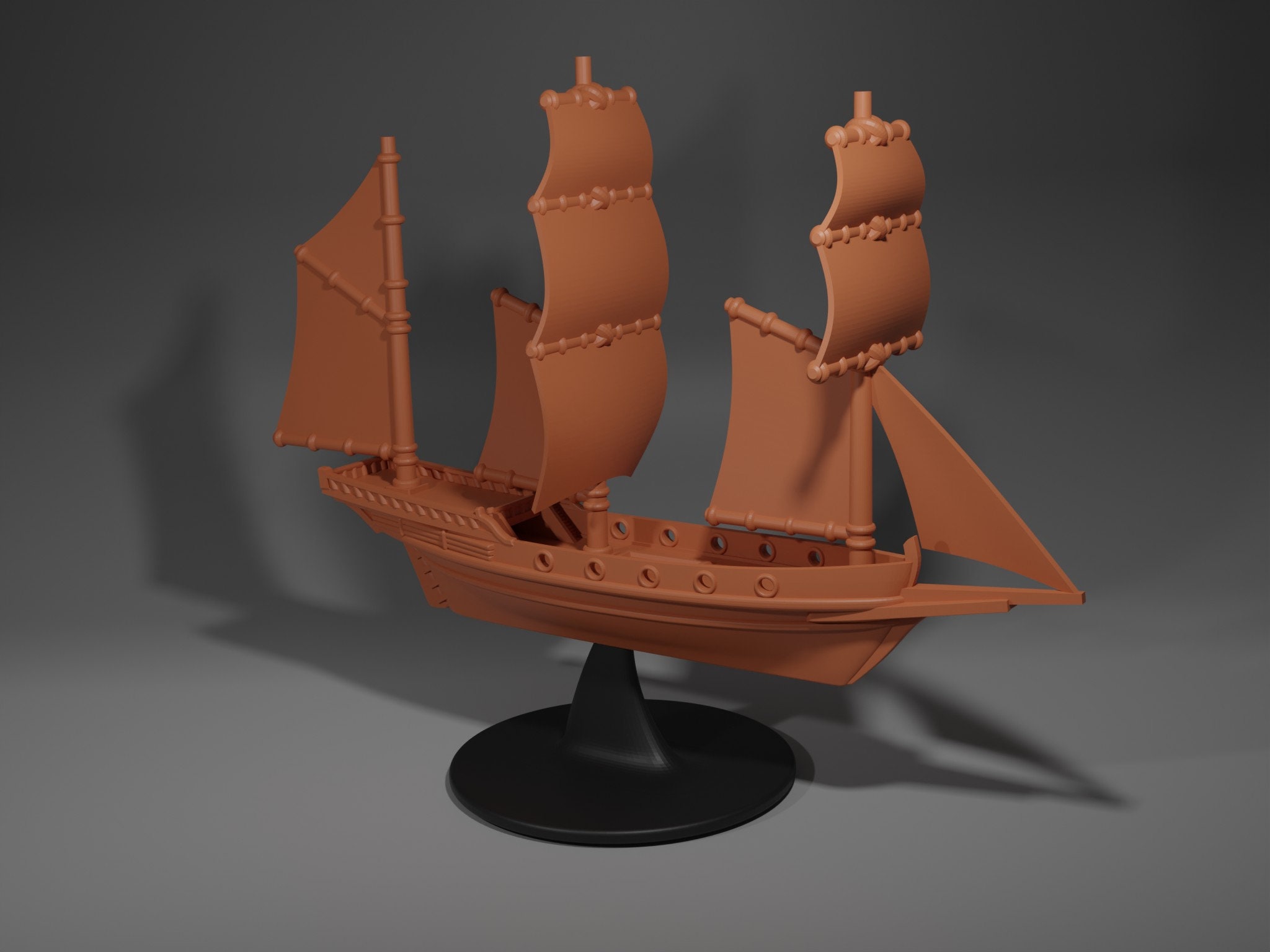The photograph showcases a meticulously crafted model of a tall ship, rendered in a light brown hue that suggests it could be made from plastic, resin, or clay. The uniform color extends across the entire model, lending it a smooth and cohesive appearance. The ship features a prominent central mast and an equally large sail on the bow, accompanied by holes along the sides where oars might typically protrude, albeit with minimal intricate detailing. The vessel is perched on a sleek black stand, consisting of a flat, round base with a triangular support connecting to the ship. This setup is set against a gradient background transitioning from dark grey to light grey, subtly illuminated from the front, which casts a distinct shadow of the ship, enhancing the overall visual depth of the image.